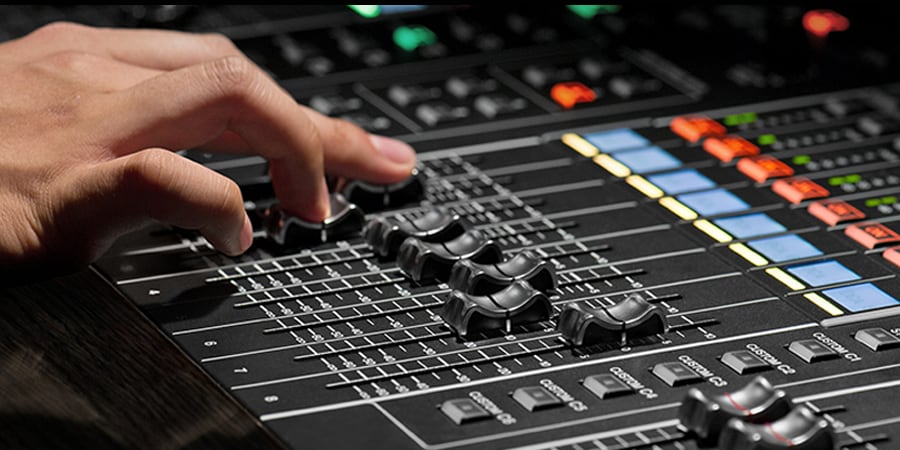This is a detailed close-up view of someone's hand operating a flat mixing table, likely in a recording studio. The image captures the hand emerging from the upper left side, manipulating three different sets of finger-shaped sliding black buttons that ride along dashed white lines marked with numbers. The mixing table features a variety of other control elements: at the very top, green and orange illuminating lights, followed by a row of flat blue buttons and smaller white and black buttons. Below these are additional gray buttons and more sliding levers arranged in descending rows. The backdrop of the photo is predominantly black with a metallic finish, adorned with a plethora of buttons and illuminated indicators. The hand, which appears to be slender and likely male, uses the middle and forefinger to adjust the sliders, suggesting active control of sound elements. The overall scene is slightly blurry in the background, highlighting the array of green and orange lights across the top of the image, reinforcing the high-tech environment of a soundboard in a recording studio.